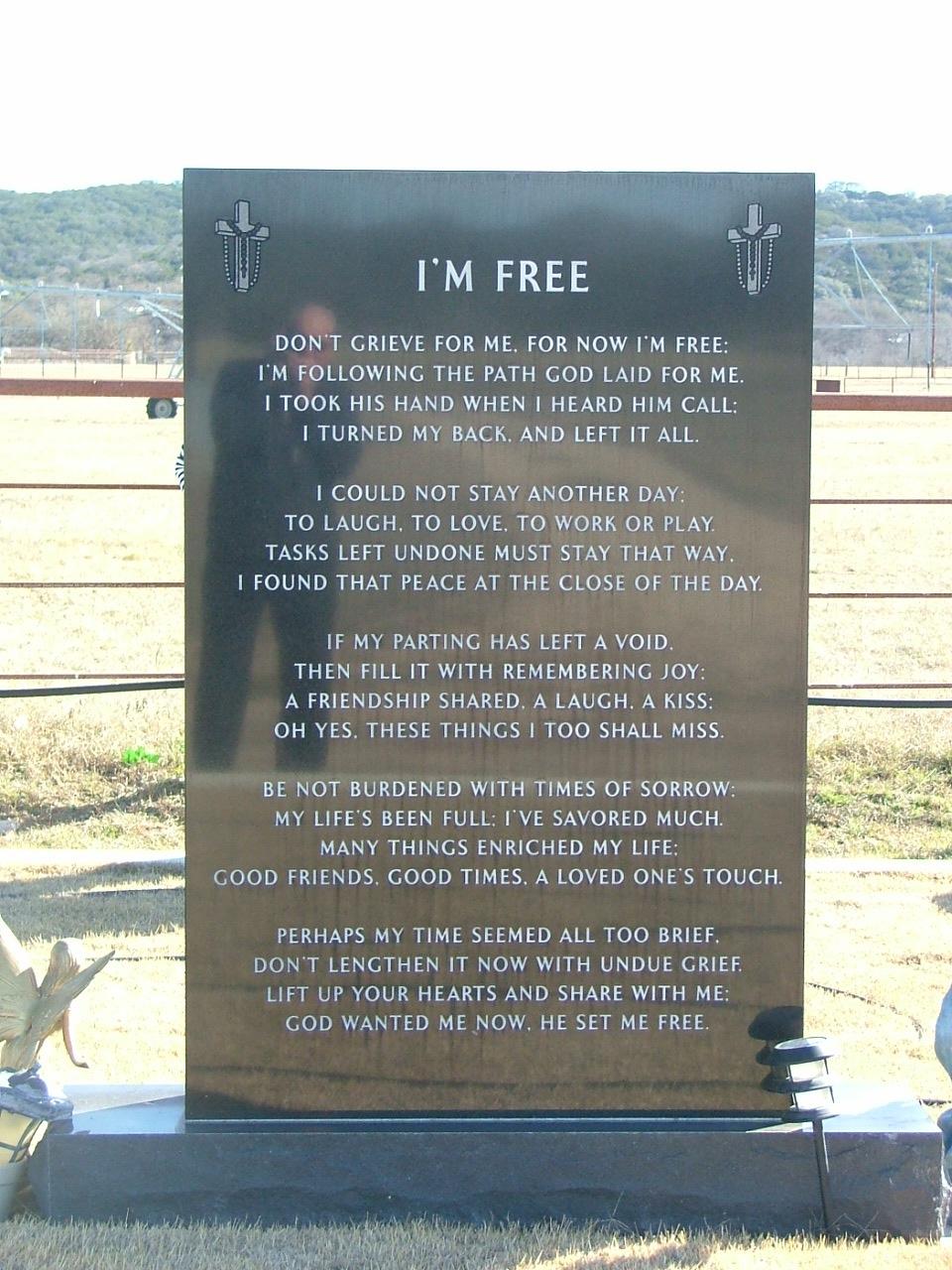In the serene countryside, against the backdrop of rolling hills and expansive farmland, stands a solemn black granite tombstone adorned with chiseled crosses and rosary beads at its top corners. The reflective surface of the tombstone captures the faint reflection of an older man, presumably the one taking the photograph. Inscribed in bold, capitalized letters at the top, the epitaph reads "I'M FREE." This poignant epitaph continues in smaller, heartfelt words:

"Don't grieve for me, for now I'm free. I'm following the path God laid for me. I took His hand when I heard Him call. I turned my back and left it all. I could not stay another day, to laugh, to love, to work or play. Tasks left undone must stay that way. I found peace at the close of the day. If my parting has left a void, then fill it with remembering joy. A friendship shared, a laugh, a kiss, oh yes, these things too I shall miss. Be not burdened with times of sorrow. My life's been full, I've savored much—good friends, good times, a loved one's touch. Perhaps my time seemed all too brief. Don't lengthen it now with undue grief. Lift up your hearts and share with me: God wanted me now, He set me free."

The text encapsulates a life well-lived and a peaceful departure, urging those left behind to find solace in joyful memories.